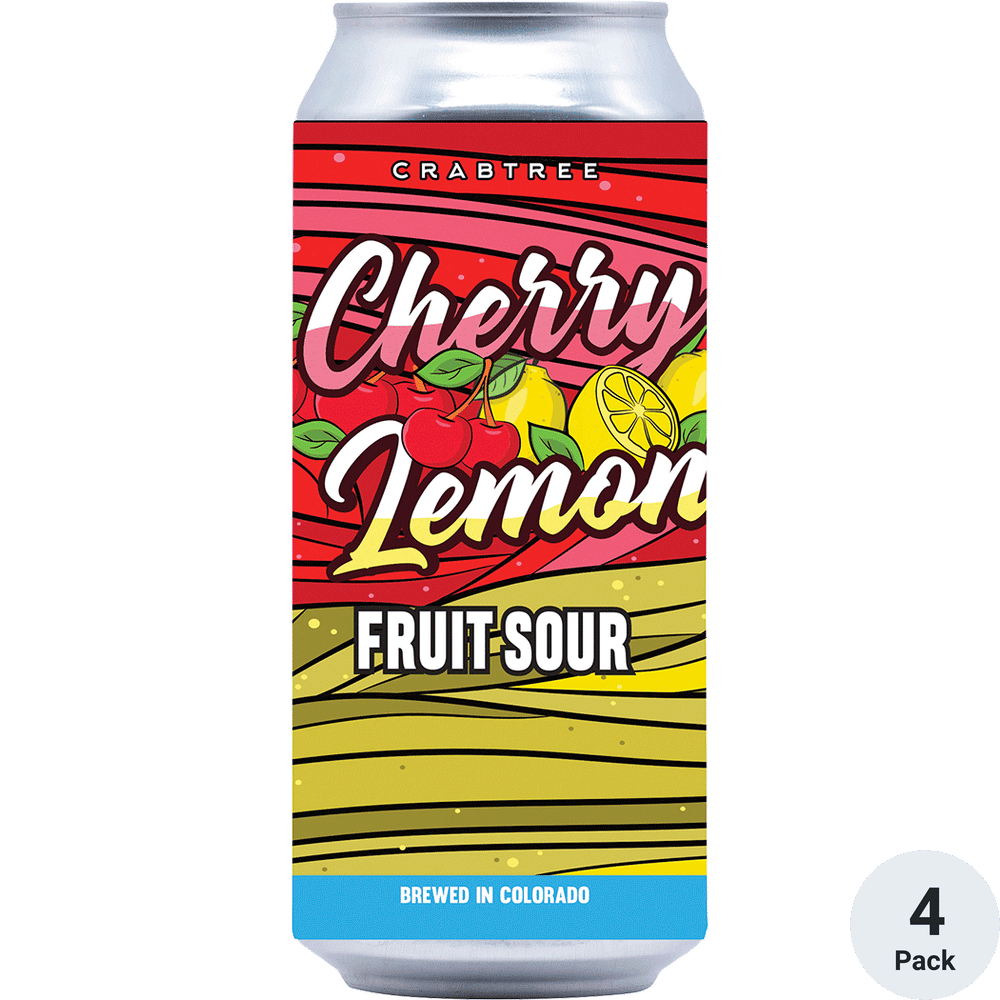The image showcases a sleek aluminum drink can set against a pure white background. The can itself occupies the entire height of the image, with a shiny chrome finish near the top where one would place their lips. The can features a vibrant, multicolored striped pattern, with the upper half in red and the lower half in green. Within the red portion, the text "Cherry Lemon" is written in script, featuring a gradient effect with light pink on the lower part of "Cherry" and light yellow on the lower part of "Lemon." This text is set at an upward angle. Surrounding the text are playful, cartoon-style illustrations of whole cherries, bunches of cherries, whole lemons, and sliced lemons. In the green portion near the border, the text "Fruit Sour" is written in all capital letters. 

At the very top of the can, in a smaller white font, it reads "Crab Tree." Along the bottom edge, the text "Brewed in Colorado" appears in white within a rectangular blue shape. In the bottom right corner adjacent to the can, a small light gray circle contains the text "4-pack."